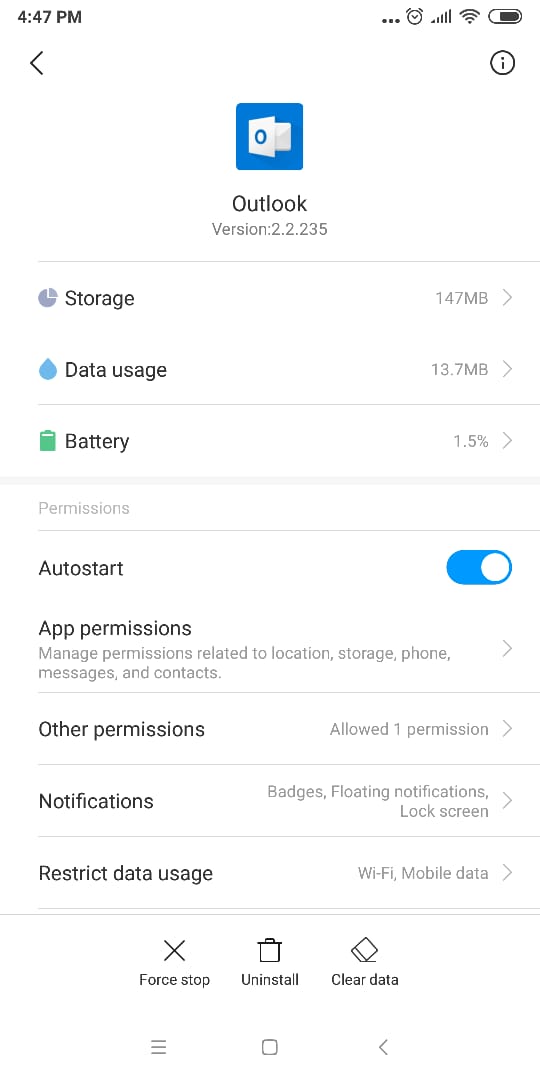The image displayed on the cell phone screen shows a detailed view of an application settings page for "Outlook." At the top of the screen, the current battery charge level is at 25% (one-quarter). The cell phone signal is strong, and the current time is 4:47 p.m. 

The web page interface prominently features the word "Outlook" in black text, positioned below a distinctive blue square emblem. Within this blue square is a white box containing a blue circle, and behind it, there’s a slightly smaller white box. 

The version of the Outlook app displayed is 2.2.235. The storage usage is 147 MB, indicated by an arrow pointing to the right for additional options. Data usage stands at 13.7 MB, also accompanied by a right-pointing arrow. The battery consumption attributed to the app is 1.5%, again with an arrow for further details.

Below these statistics, there is a section labeled "Permissions" which includes an Auto Start button that is currently toggled on, as indicated by its illuminated blue color. The "App Permissions" category allows the management of permissions related to location, storage, phone messages, and contacts. The "Other Permissions" category states that one permission is allowed.

The "Notifications" section outlines options for badges, floating notifications, lock screen settings, and restrictions on data usage via Wi-Fi and mobile data.

At the bottom of the settings page, there are three actionable buttons: "Force Stop," "Uninstall," and "Clear Data."